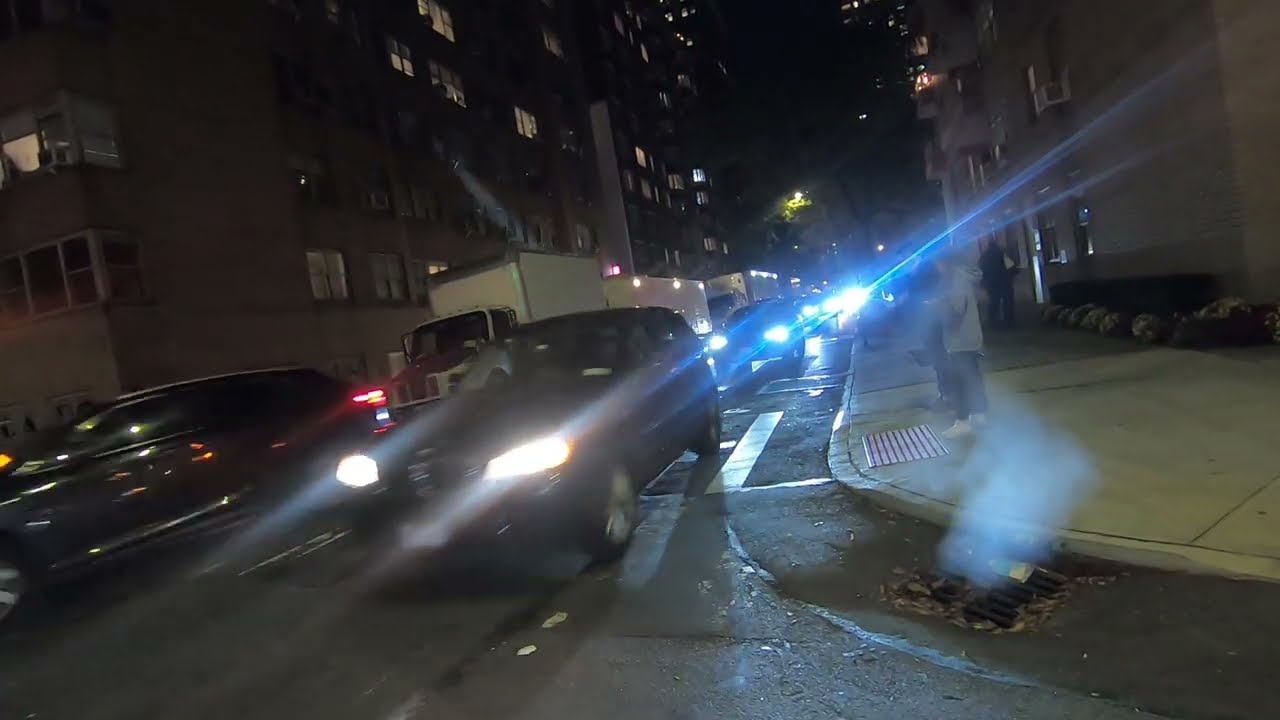This nighttime city scene captures a bustling street filled with various vehicles, including a blurred car in motion, dark subcompacts, sizable white trucks, and SUVs, all with their headlights on. The street, which appears to have at least two lanes of heavy traffic, runs through an intersection, clearly indicated by a visible crosswalk and the curve of the sidewalk on the right. Steam is rising from a grate in the street, adding to the urban atmosphere. Pedestrians are present; one person is walking along the sidewalk while a couple of others stand waiting to cross. The background is lined with tall buildings, possibly residential apartments, that span at least three to four stories high. The building windows are a mix of lit and dark, with so many lights that they cause an artifact of light beams and a glare in the image. This photograph, despite being slightly blurry, vividly depicts the lively and dynamic essence of a city street at night.